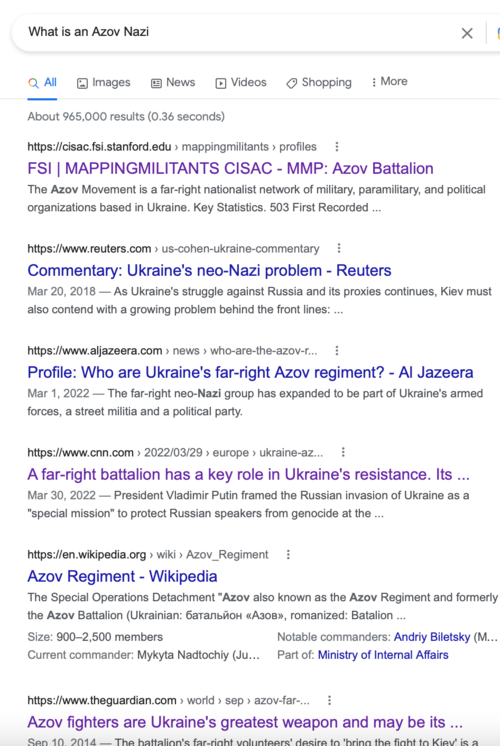A cropped screenshot of a Google search is displayed, focusing on the search results. At the top of the image, the search query "what is an Azov Nazi" is visible in small black font inside the search bar located on the left side. The right side of the search bar, including the Google logo and microphone icon, is not visible due to cropping. Six categories—All, Images, News, Videos, Shopping, and More—are horizontally aligned below the search box. The search results show that the first, fourth, and sixth links have been clicked, as indicated by their purple color. The remaining links are blue, signifying they are unclicked. The results are cropped so that only the top portion of the sixth entry is visible, and additional elements of the page are not included in the screenshot.